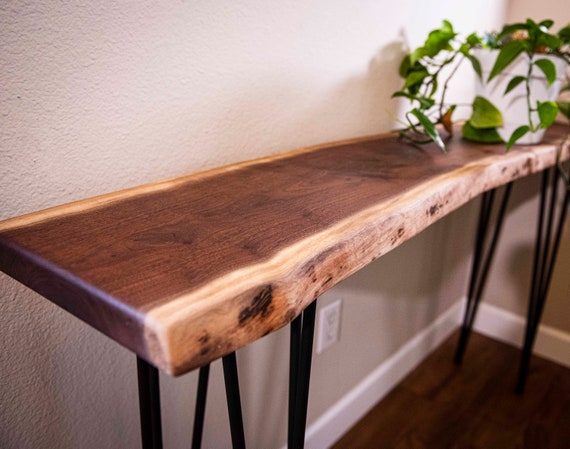The image features an indoor setting with a hardwood floor, brown in color, that stretches across the ground surface. Against the background, there is a textured off-white wall to the left and a white wall to the right. At the intersection where the two walls meet, a table or a stand is positioned directly in the center of the image. The table, which anchors the composition, has a wooden top, and its brown surface reveals a distinct wood grain. Supported by black, triangular-shaped legs, the table spans from the left center of the picture to the top right corner. A white flower vase sits near the upper right corner of the table, holding a green plant with noticeable leaves and stems. Below the table, mounted on the white wall, is a black electrical socket. The colors in the scene include various shades of brown, tan, beige, green, light green, white, and black. The focus seems sharper on the left side of the image while the right side appears slightly blurred. The photo captures an indoor space, possibly within someone’s home, and does not contain any text or indicate the time of day.